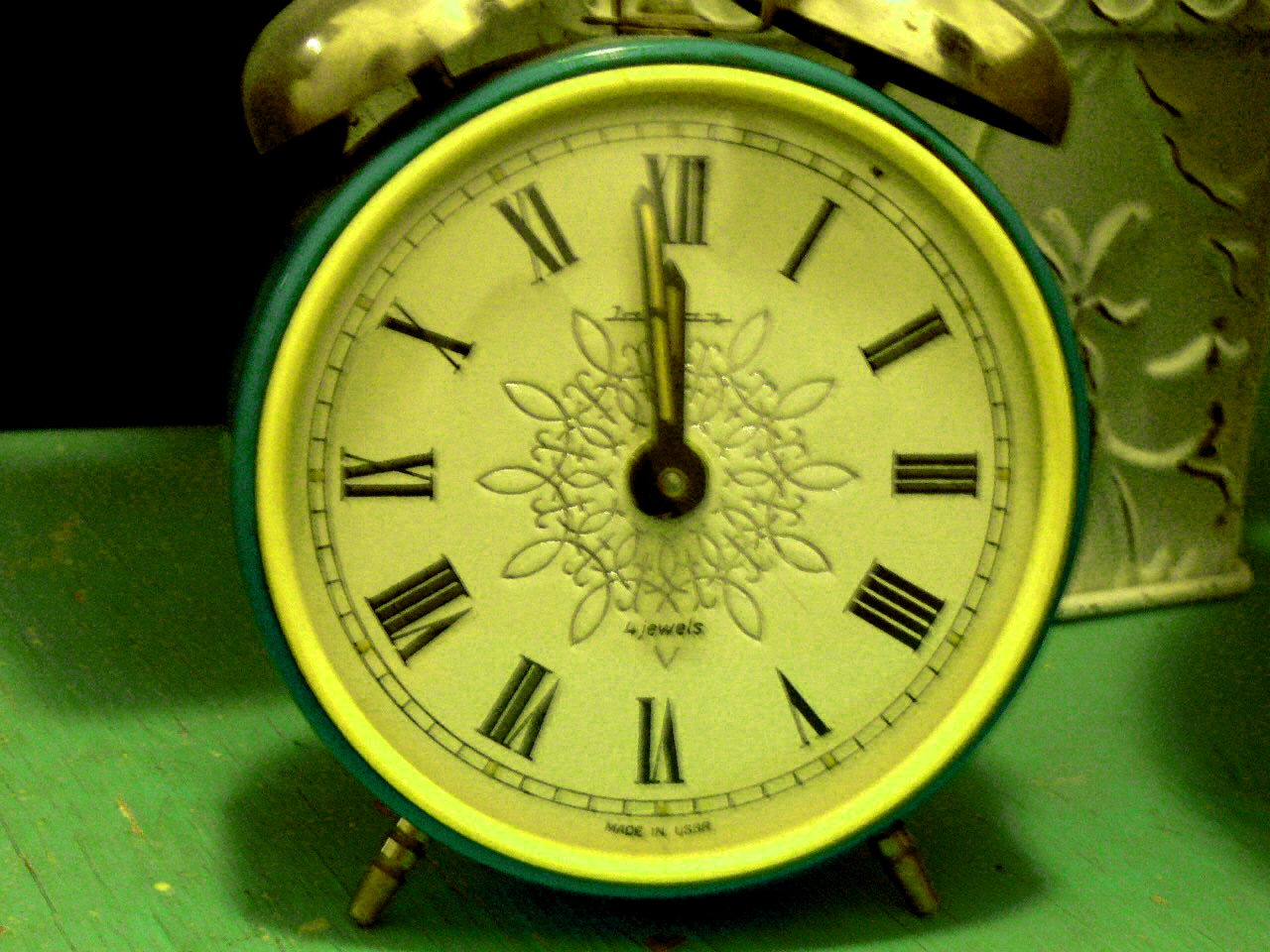The photograph, taken indoors, centers on a vintage-style alarm clock, framed by a black background that accentuates its detailed features. The alarm clock, resting on a weathered green-painted wooden table, commands attention with its distinctive green metal exterior and golden auditory bells perched atop. The clock stands firmly on two gold-toned legs, adding to its antique charm. Behind the timepiece, a metallic green object can be partially seen, though it remains largely hidden by the clock.

The clock face is a stark white canvas, adorned with bold black numerals that stand out clearly. The clock's hands – mostly black with subtle yellow stripes – are poised in precision, hinting at the meticulous craftsmanship. At the center of the clock face, a delicate pattern catches the eye, along with the inscription "Four Jewels." The bottom of the clock proudly declares its origin with the words "Made in the USA," further emphasizing its historical significance and quality craftsmanship.